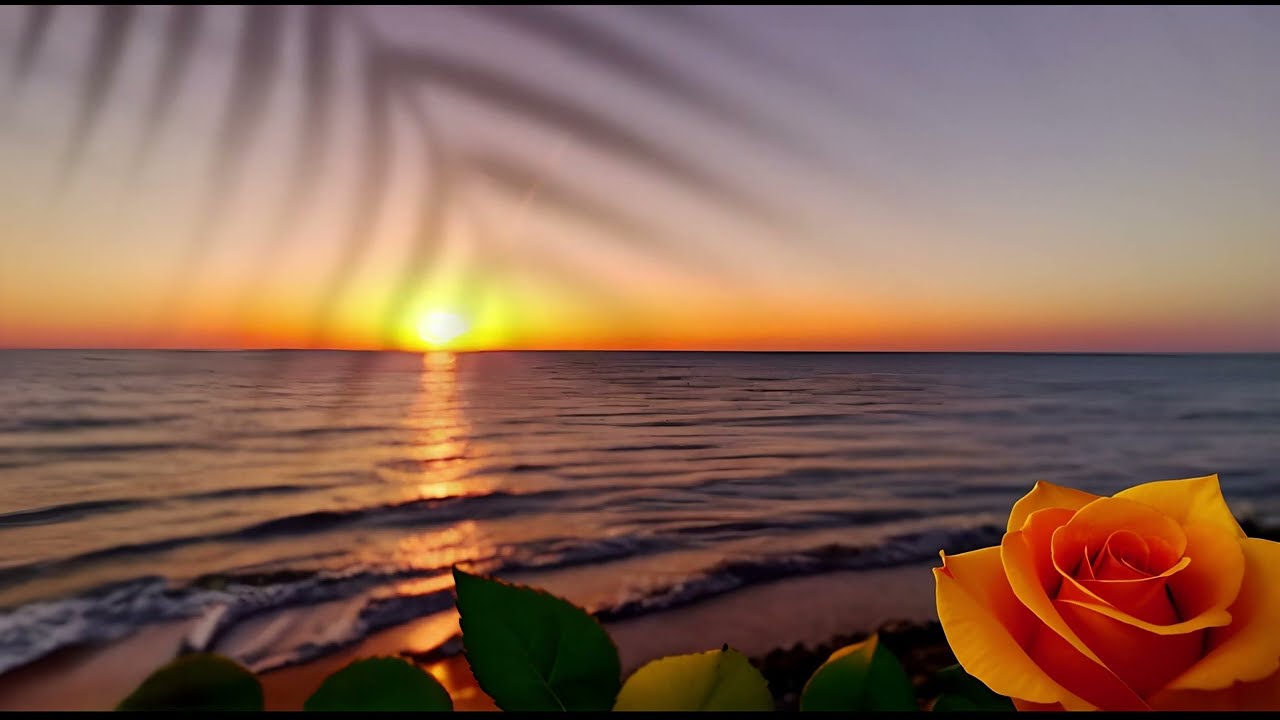As the sun sets on the horizon, the scene is bathed in an array of stunning colors. The central circular white sun, encircled by a halo of yellow, is just touching the sea, creating a brilliant yellow gleam on the light dark blue ocean, adorned with gentle waves. The sky transitions from yellow near the horizon to a purplish-gray at the top, showcasing the last light of day. This evocative image, whether a photograph or a painting, captures a tropical setting with remarkable detail. In the foreground, to the lower left, delicate green palm leaves extend into the frame, and on the bottom right, a sharply focused orange rose adds a vibrant contrast. The sky and ocean, slightly out of focus, highlight the sharpness of the leaves and flower, enhancing the depth of this picturesque scene.